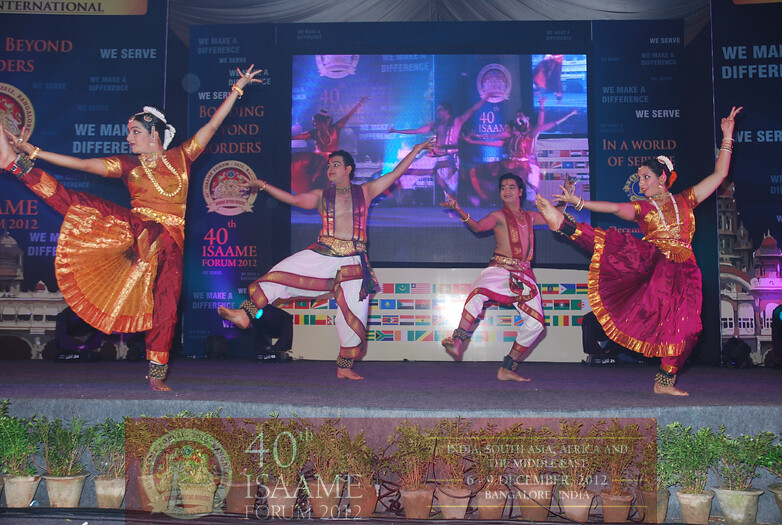The image captures a vibrant cultural event featuring a South Asian dance performance on stage at the 40th ISAM Forum 2012. Four dancers are striking a synchronized pose, with two women on the far left and far right wearing ornate traditional attire, comprising red or purple pants with a golden-red top and a flowing front skirt. The two men positioned between them adorn white flowy pants with red and gold trim. All four dancers are barefoot. The stage is adorned with several potted plants in tan-colored pots, adding to the cultural ambiance. Behind the dancers, there's a screen displaying their live image, and flanking the screen are inspirational phrases like "In a world we serve," "We make a difference," and "Going beyond borders." Additional flags from various countries are visible on a white sheet below the screen, possibly representing the international nature of the event.